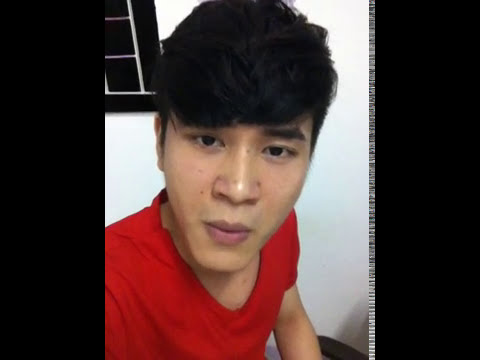This image depicts a young Asian man, likely in his 20s or 30s, taking a selfie. He has black hair and is wearing a red v-neck t-shirt. He is seated and looking straight into the camera with a neutral expression, not smiling. One of his hands is partially visible, presumably holding the camera. The background features a white wall and a black window with white grills on the top left-hand side, adding minimalistic elements to the otherwise simple scene.